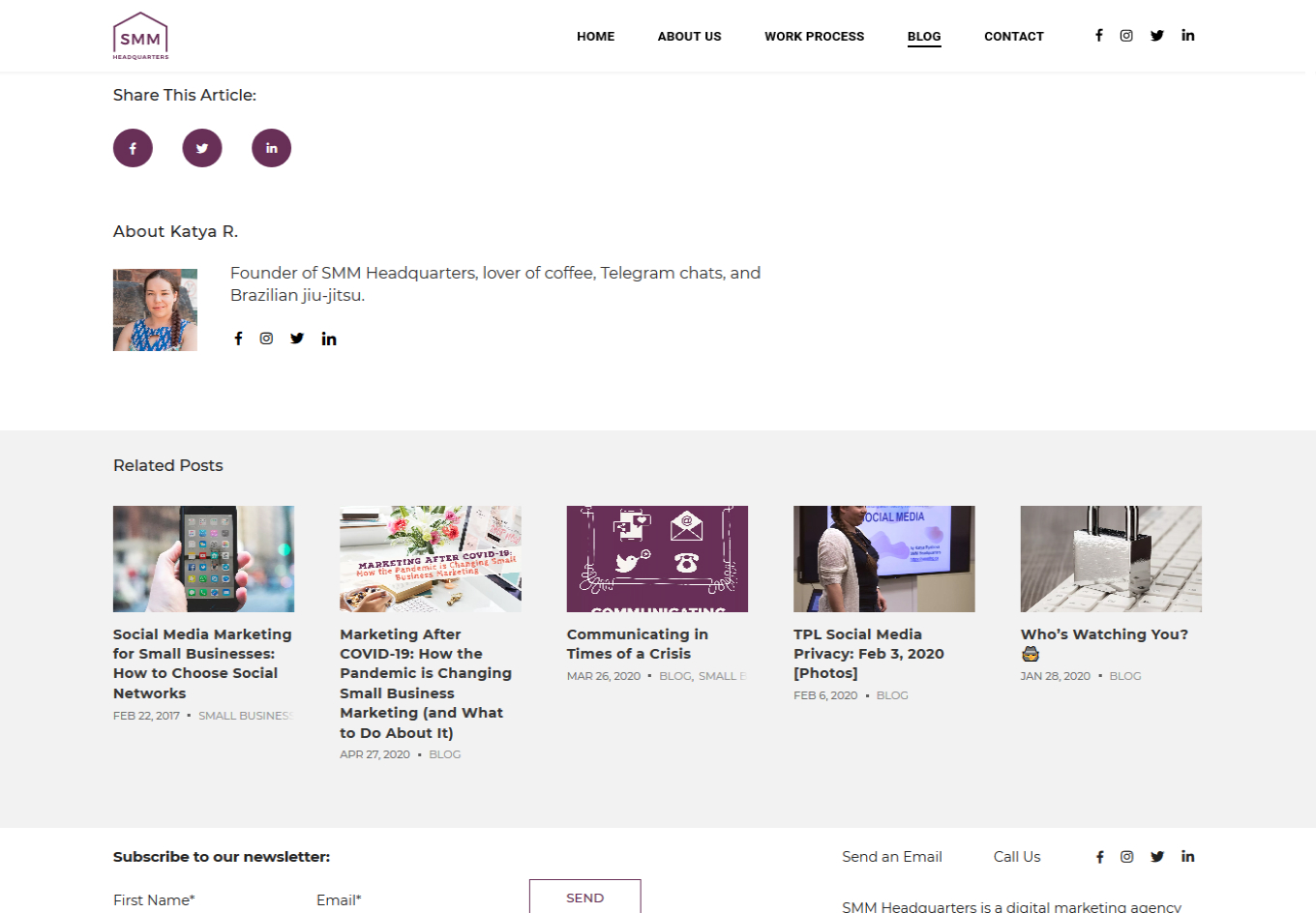Caption: 

The image is set against a white background featuring a central visual of a purple house. Prominently displayed in capital letters are the initials "FMN" in purple. Below this heading, red underlined text includes links to sections titled "Home," "About Us," "Work," "Process," and "Blog." The "Contact" section is accompanied by icons for Facebook, Twitter, Snapchat, and LinkedIn.

Further down, a segment invites users to "Share This Article," with three circular icons for Facebook, Twitter, and LinkedIn. There is a detailed "About Katar" section which includes a picture of Katar, who is described as the founder of SMM Headquarters and a lover of coffee, Telegram chats, and Brazilian jiu-jitsu (spelled out as j-i-u j-i-t-s-u). This section also features icons for Facebook, Snapchat, Twitter, and LinkedIn.

Additionally, there are five related articles listed:
1. "Social Media Marketing for Small Businesses"
2. "How to Choose Social Networks: Marketing After COVID-19"
3. "How the Pandemic is Changing Small Businesses" (noted as "Small Business Marketing")
4. "What to Do About It: Communicating in Times of Crisis"
5. "TPL Social Media Privacy" dated February 3rd, 2020, with accompanying photos.